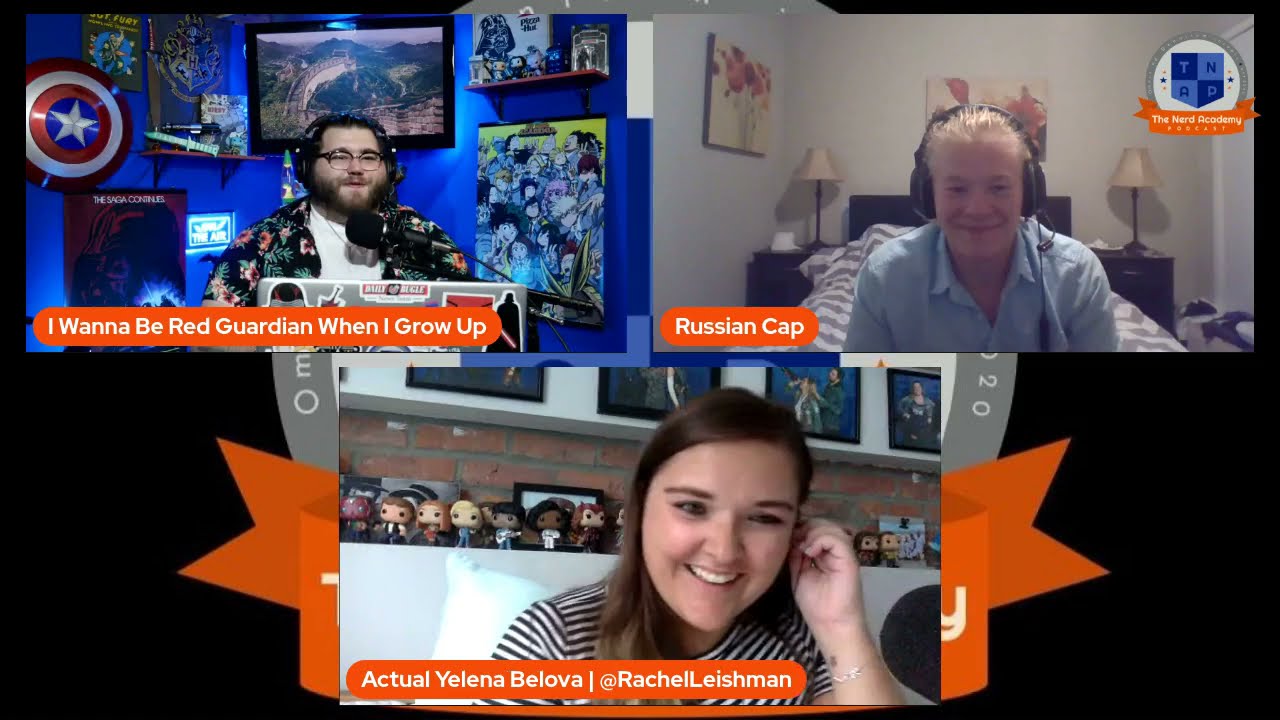The image depicts a video conference call with three participants in separate frames. The two frames at the top show two men, while the bottom frame features a woman. The top left frame presents a white man with short hair, a beard, and glasses, wearing a black Hawaiian shirt with flowers. He is sitting in front of a sophisticated microphone setup, with a room filled with comic book memorabilia, including a Captain America shield, and Star Wars and Harry Potter items. His caption reads, "I want to be Red Guardian when I grow up."

The top right frame features another white man with spiky, beach-blonde hair, wearing black over-the-ear headphones and a blue button-down shirt. He appears to be in his bedroom, with a bed that has a gray and white striped comforter and black headboard. His caption is "Russian cap."

The bottom frame shows a white woman with long brown hair, wearing a black-and-white striped shirt. She is seated at a desk with shelves behind her filled with Funko Pop figures and a brick wall in the background. Her caption states "actual Yelena Belova" with her handle "@RachelLeishman." The video call seems to be hosted on a platform, possibly StreamYard, under the banner "Nerd Academy," suggesting a discussion on nerd culture or related topics.